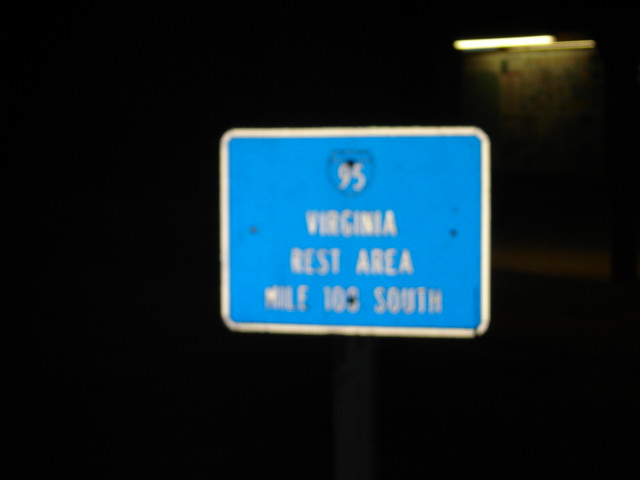A captivating night-time photograph captures a somewhat blurred blue road sign, edged with reflective white. At the top center of the sign, a distinctive root symbol frames the number "95." Beneath the root symbol, the sign reads "Virginia" in clear white letters. Following this, "Rest Area" is prominently displayed, with the notation "Mile 101 South" below it. The photograph's background is enveloped in deep darkness, emphasizing the night-time setting. In the upper right corner of the image, a lone horizontal fluorescent light hovers, likely from a building, suggesting the proximity of the actual rest area. The stark contrast between the illuminated sign and the encroaching night sky creates a visually intriguing scene.